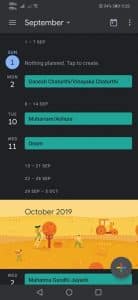The image displays a smartphone screen with a calendar app open. The upper portion of the screen has a black background. The calendar app is currently displaying the month of September. The date "September 1" is highlighted in blue. Several dates have highlighted plans: the 2nd, 10th, and 11th of September, each marked with a green background. The text detailing these plans is written in black but appears blurry and unreadable.

At the bottom of the screen, the following month, October 2020, is displayed. The background for October 2020 is orange and adorned with seasonal drawings. On the right side, there is an illustration of a tractor or car, next to a person walking a dog near a tree featuring brown and orange leaves. There is also a plan marked on October 2nd.